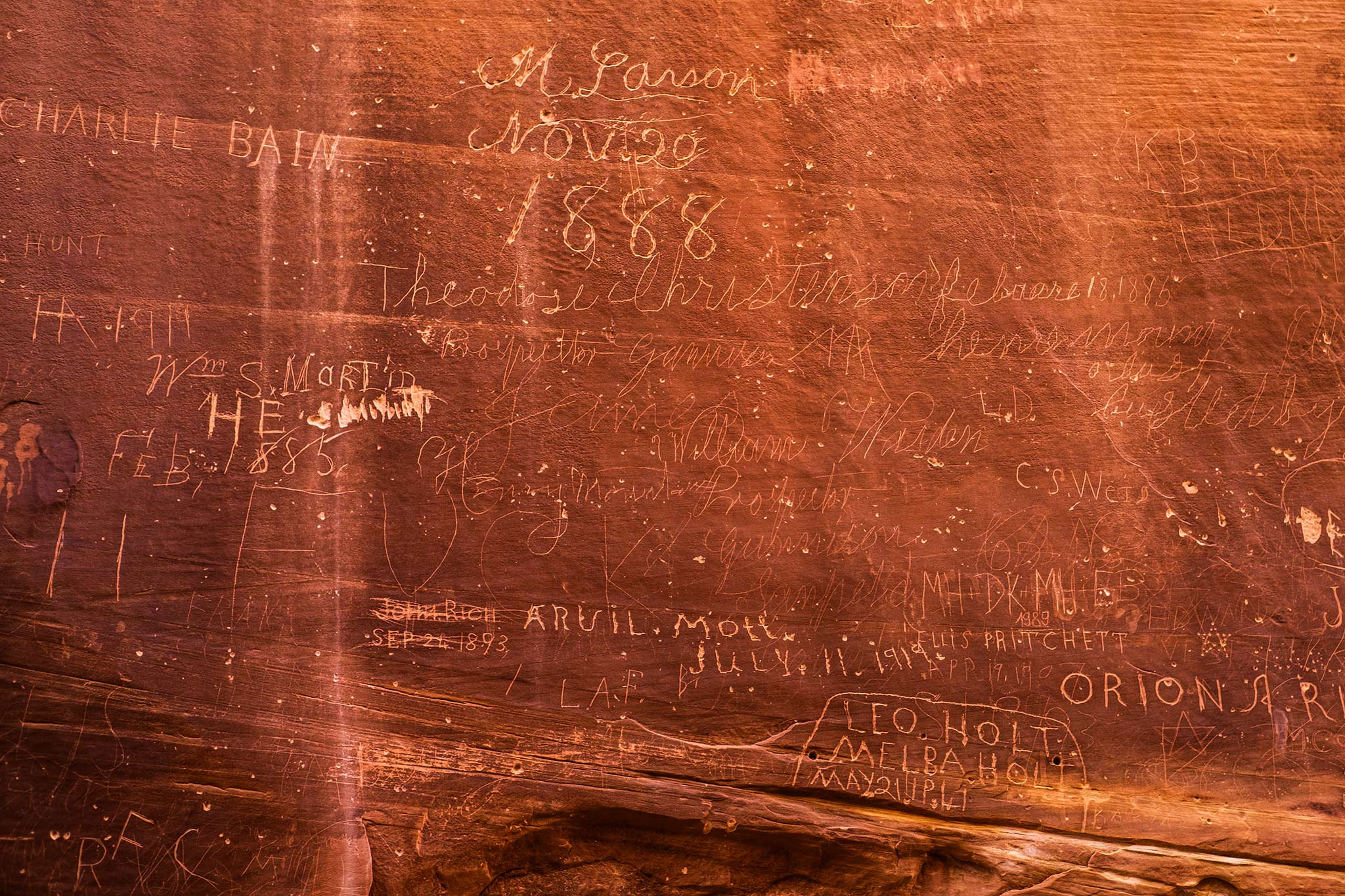The image depicts a reddish-golden, weathered wall that might be made of stone or wood, featuring an intricate texture with ridges that resemble natural materials. The surface is etched with various names and dates in different handwriting styles, suggesting a long history. Among the carvings are notable entries such as "Charlie Bain, 1888," "Leo Holt, February 1885," "Melville Holt, May 21st," and "Orion of Vermont, July 11th, 1919." The wall exhibits signs of wear and tear, with some areas worn down and a significant chunk missing near the lower section. Scattered across the wall are random, scratched-on letters and numbers, adding to the aged and rustic appearance. The coppery hue of the wall is highlighted by occasional light reflections, enhancing its textured, antiquated look.